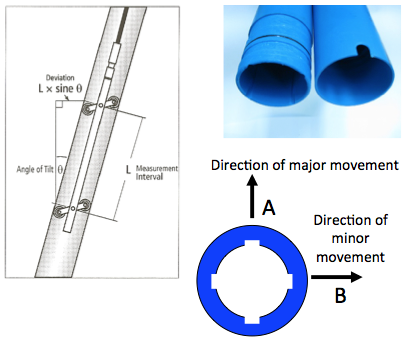The infographic presents a detailed diagram and photograph of a mechanical component against a white background. On the left side, inside a thinly outlined gray rectangle, there is a vertical cross-section of a tube housing a metal rod with two wheeled mechanisms. The diagram includes mathematical notations such as "Deviation L × sin(θ)" and labels indicating "Angle of Tilt." Measurement intervals are marked between the mechanisms within the tube.

On the right side, the upper quadrant features a photograph of two blue plastic tubes, one with a threaded end and the other notched, set against a white and blue background. Below this, the bottom right quadrant showcases a simplified cartoonish cutaway of the tube with directional annotations. The annotations indicate "Direction of Major Movement" with an arrow pointing upward labeled 'A', and "Direction of Minor Movement" with an arrow pointing to the right labeled 'B'. This detailed composition effectively illustrates the components and their functions.